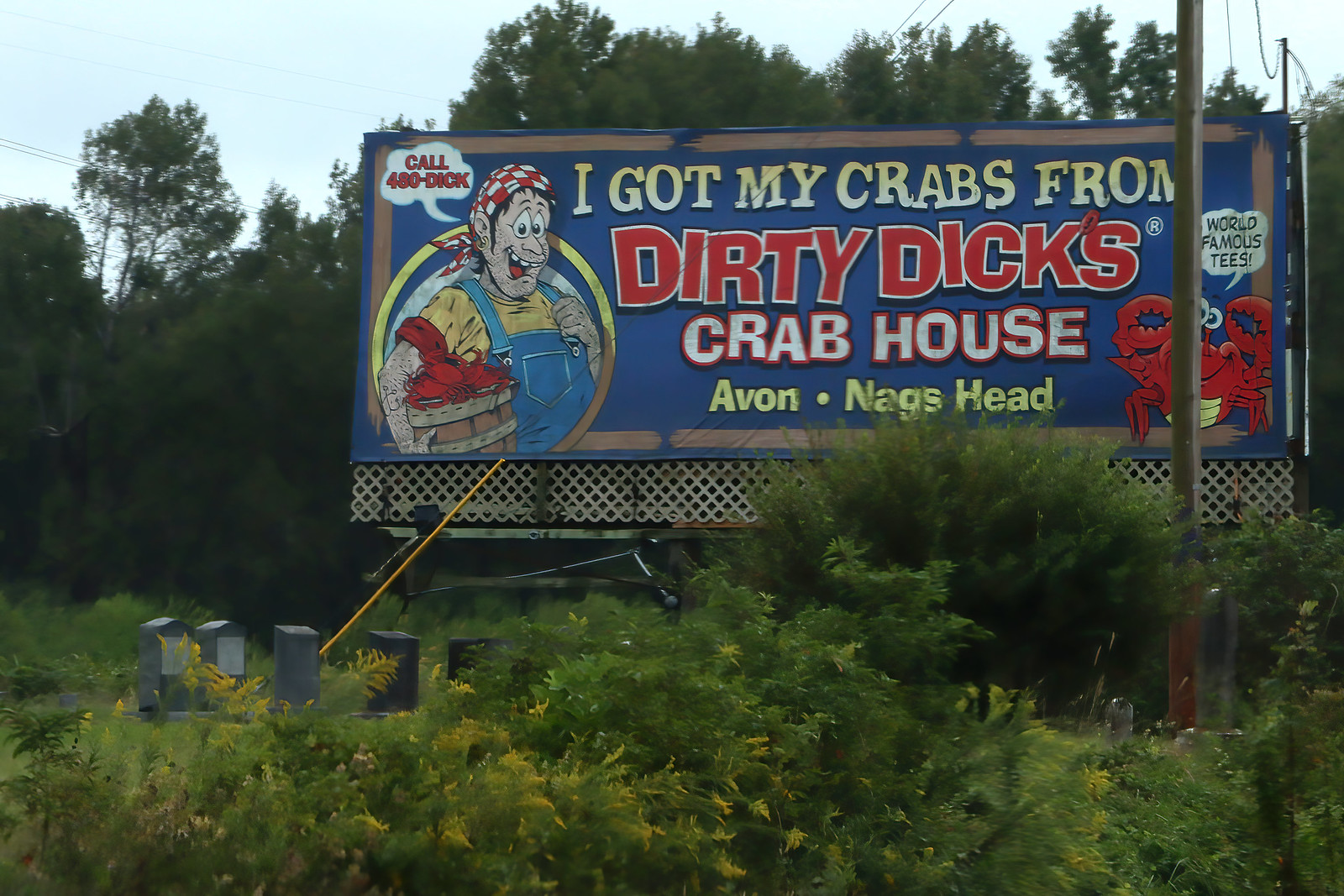This photograph captures a large billboard prominently displayed alongside a road, with a background featuring tall green trees and a light grayish-blue sky. The billboard is predominantly blue, trimmed in brown, and supported by a metal stand. It stands elevated above some bushes, a gray and black fence, and there are telephone poles and wires nearby.

The text on the billboard reads in sequence: "I got my crabs from" in yellow at the top, followed by "Dirty Dicks" in bold red, and "Crab House" in white with a red outline. Below this, "Avon Nags Head" is written in yellow, highlighting the two locations.

To the left side of the billboard, there is a cartoon depiction of a Caucasian man, designed to look like a comical hillbilly. He has exaggerated features including big eyes, prominent buck teeth, a wide smile revealing a red tongue, and short black hair. He wears a red and white checkered bandana tied around his head, a yellow t-shirt, and blue overalls. The character is humorously holding a brown basket filled with red crabs. Above the character is a speech bubble in white saying, "Call 480-DICK."

Additionally, the bottom left corner of the billboard features a red crab with beady white eyes and blue pupils, emerging from the blue background. Above the crab is a white speech bubble stating, "World Famous Tees!” with an exclamation point.

In the surroundings, there are some gray and black headstones to the left of the billboard, which adds a peculiar touch to the overall scene. The photograph has a bright, clear atmosphere, amplifying the vibrancy of the billboard’s colors.